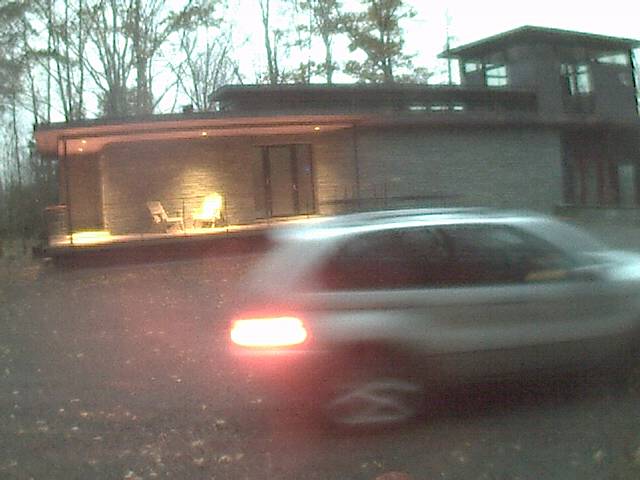A blurry nighttime photograph depicts a gray sedan, possibly a hatchback, parked outside a building or house. The car’s taillights are illuminated, and an indistinguishable arm appears to be adjusting the side rearview mirror. The ground, covered in a scattering of leaves, is predominantly gray. 

The building is rectangular, featuring a porch on the left side adorned with a set of chairs facing each other under the glow of a porch light. The right side appears to be under construction, with multiple openings suggesting unfinished walls or structures.

The sky suggests it is evening, around 7 or 8 o'clock, and in the background, you can see silhouettes of trees with sparse, dark brown leaves. The house is primarily constructed of gray horizontal bricks, with the right side having a higher section with exposed openings, adding to the impression of ongoing construction.